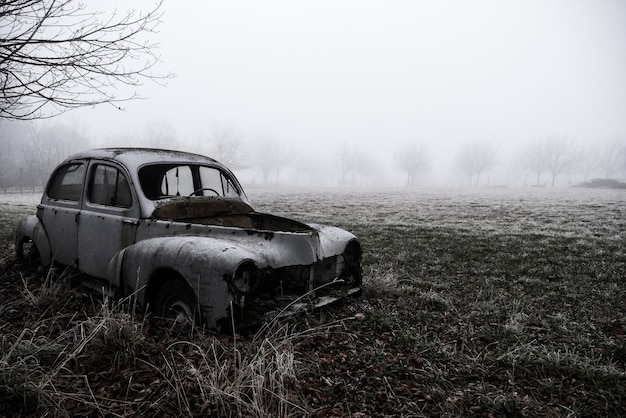In this haunting black and white photograph, a desolate, ruined car sits abandoned in an empty, dark field. Shrouded in thick fog, the background reveals a hint of leafless trees dispersed across the horizon, enhancing the eerie atmosphere of the scene. The sky above is a pale, hazy gray, blending almost seamlessly with the foggy backdrop. On the upper left edge of the image, stark black branches stretch out from a dead tree, devoid of any foliage, a stark indication of winter's touch.

The central subject, an old, rusted car, appears heavily distressed and neglected. Its hood and headlights are missing, revealing a dark, rust-eaten body that merges into the monochrome tones of the image. The car lacks a bumper and wheels, emphasizing its abandonment. Surrounding the car, patches of white-tinted grass and dark dirt add to the sense of desolation. The lower portion of the field features long, unkempt weeds in the left corner, with slightly shorter grass spreading out across the center. The car is positioned slightly to the left and angled towards the lower right corner, completing this stark and evocative scene.